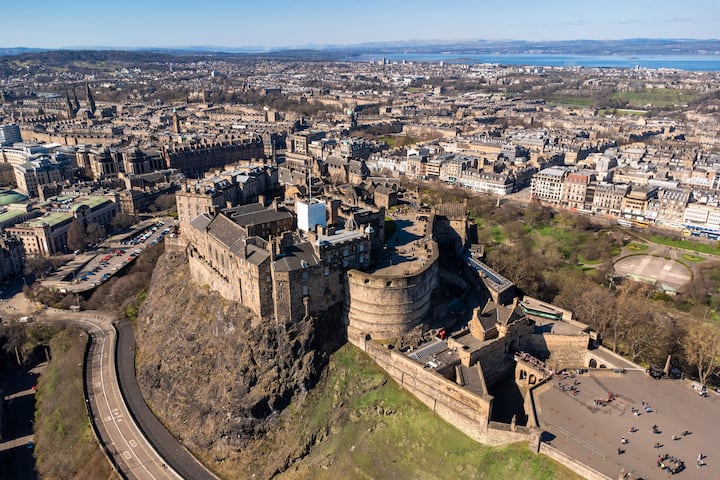This aerial view captures a historically significant site prominently perched on a rocky hilltop, surrounded by a bustling urban landscape. The central focus is an imposing old palace or castle, characterized by its high protective walls and fort-like structure, a relic from bygone times designed for defense. The fortress is now a popular tourist destination, evident from the visitors walking across a bridge leading from a large parking lot into the vast palace grounds.

The scene extends to a densely populated city, abundant with high-rise buildings and lacking in residential houses. Beyond the urban sprawl, the horizon reveals a serene expanse of water, providing a picturesque backdrop along with a smattering of green fields and trees, suggesting a lush spring or summer setting. A highway encircles the castle-topped hill, adding to the modernity juxtaposed against the historical edifice. The aerial shot, likely captured by a drone, encapsulates a vivid blend of ancient architecture and contemporary city life, evoking a European, possibly Iberian, ambiance.